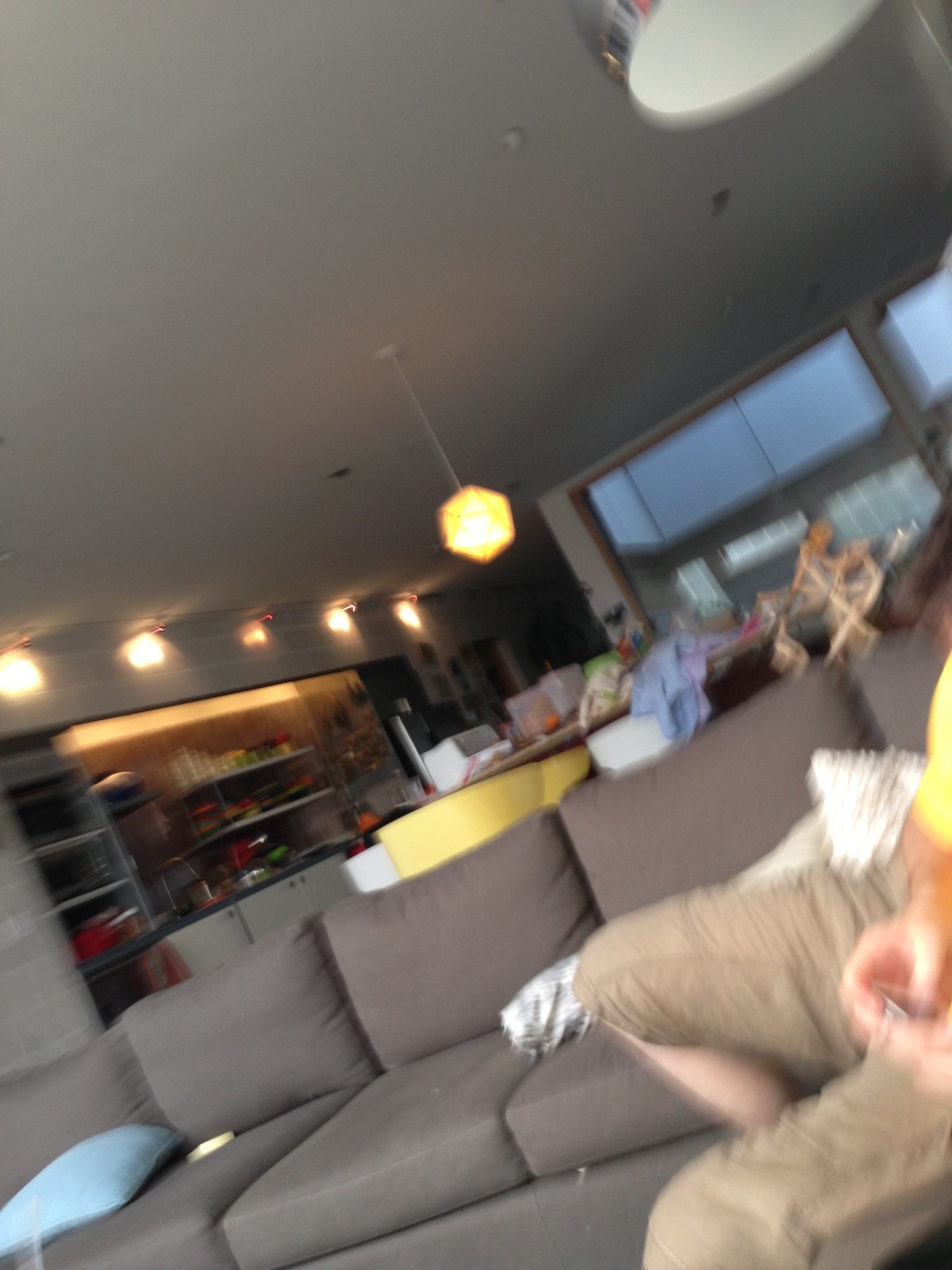This photograph captures a cozy and modern living space inside a home, presenting a detailed look at both the living room and the adjoining kitchen. On the right side of the image, a person's arm, clad in a yellow sleeve, extends into view as they manipulate a cell phone. The individual, who is wearing khaki-colored cargo shorts, is seated on a dark gray sectional sofa adorned with several cushions - white, black, and a blue pillow in the distance. 

The background reveals a kitchen area characterized by a blend of yellow and white chairs encircling a cluttered kitchen island. This island holds assorted items, including blue and purple fabrics—possibly rags or clothing—and various containers, contributing to a lived-in feel. The kitchen is bathed in a warm glow from a bright yellow pendant light hanging from the ceiling. On the left, white cabinets and gray tiled backsplash set a neutral tone, while five distinct lights illuminate the kitchen area. Various open containers and items are visible, adding to the room's everyday practical aesthetic.